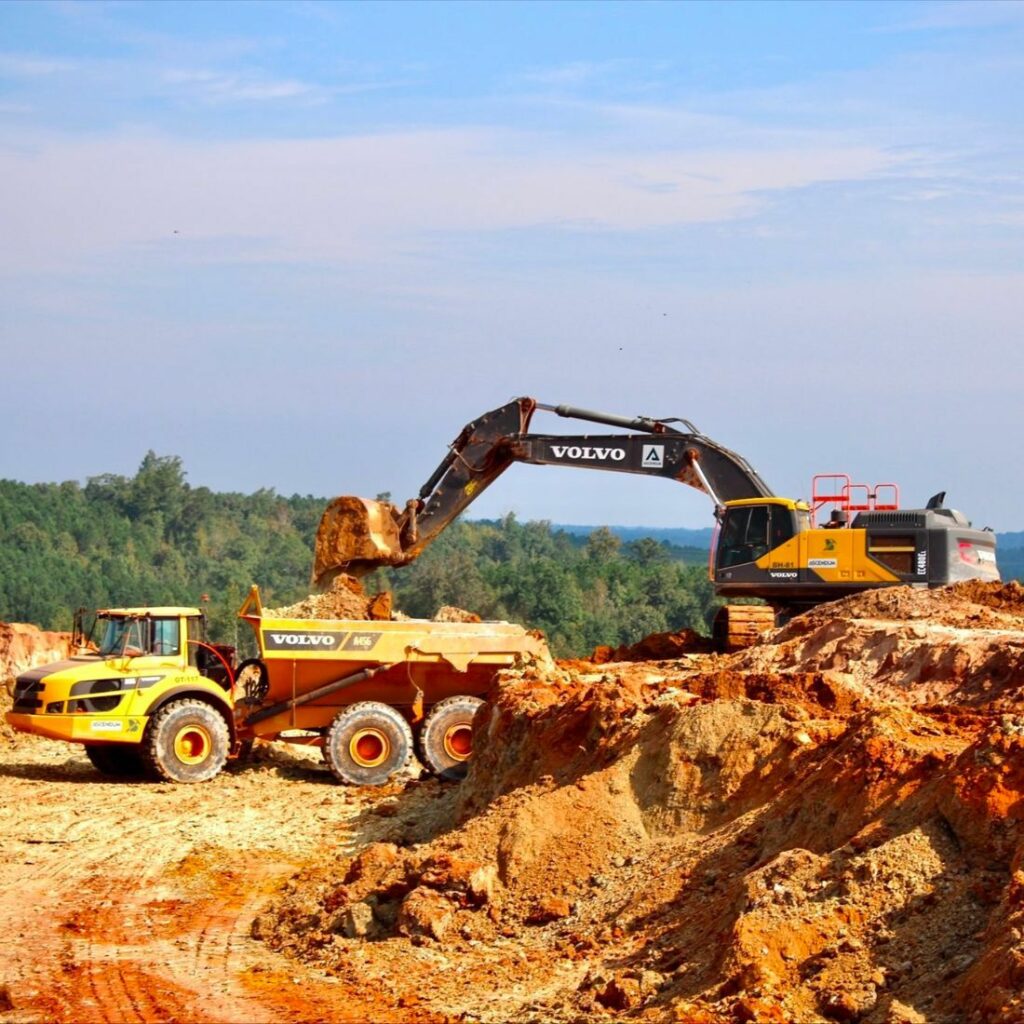In this detailed image of an excavation site, a yellow and black excavator labeled "Volvo" is seen actively dumping dirt into the bed of a yellow dump truck, also marked with the Volvo brand. The machinery is situated on a rough, dry landscape of orange, brown, and cream-colored soil, emphasizing a very rocky and craggy terrain. Nearby, a large mound of brown dirt, previously excavated, rests on the ground. In the distance, the background features a dense formation of evergreen trees stretching from the left to the middle of the scene, giving way to a slightly cloudy blue sky with hazy, off-white clouds tinged with a hint of lavender. The overall site combines elements of both construction and excavation, framed by the natural forestry and sky.